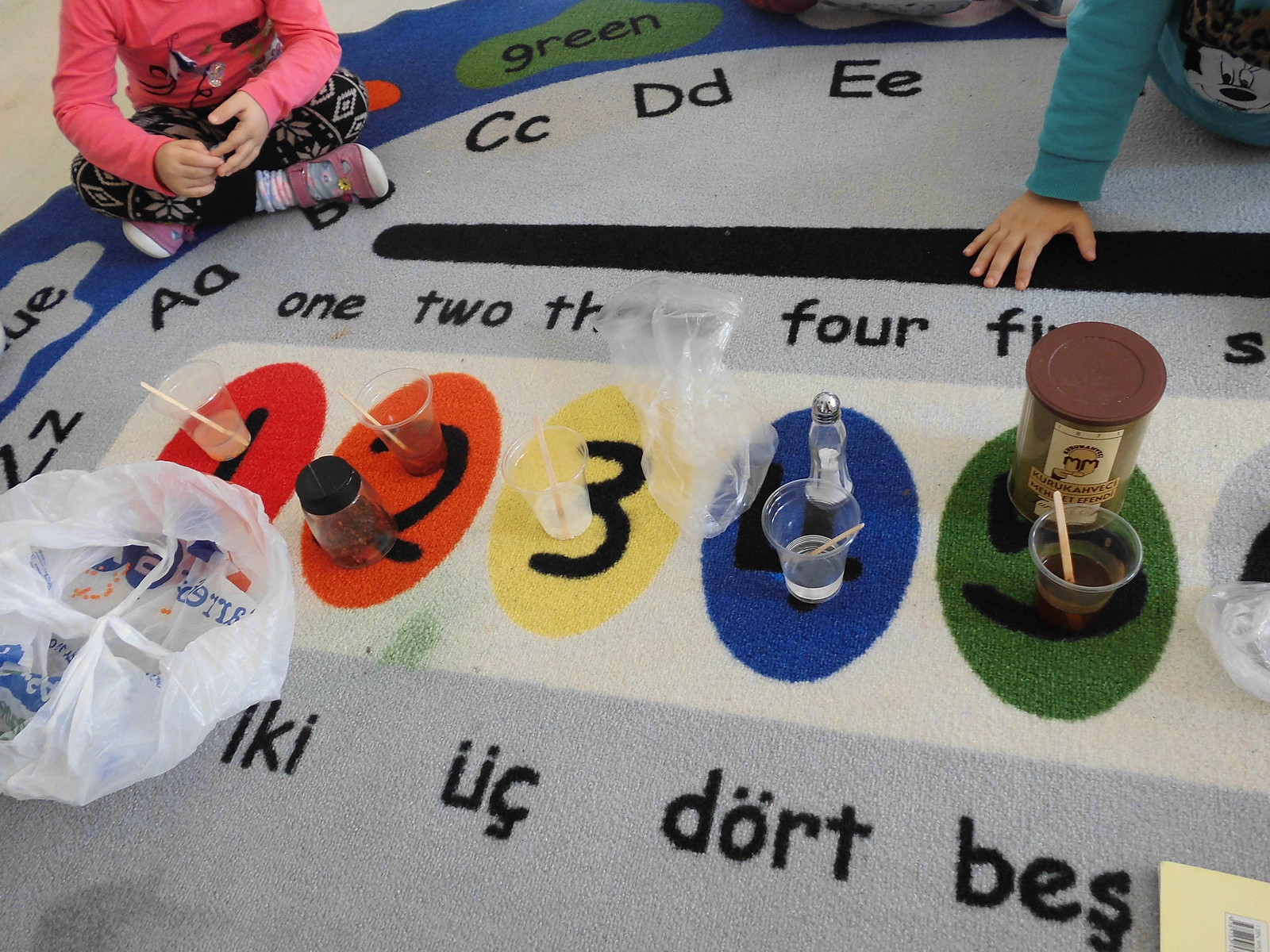The image portrays a vibrant classroom scene where children are engaged in a science experiment on a specially designed, educational rug. This rug predominantly features a gray background with a blue border and showcases the periodic table of elements around its edges. In the center, it displays six vividly colored circles arranged from left to right, each containing educational elements. 

The red circle contains the number 1, the orange circle has the number 2, the yellow circle holds the number 3, the blue circle shows the number 4, the green circle presents the number 5, and the gray circle displays the number 6. Each number is showcased in black within its respective circle. Additionally, the numbers are spelled out in text above and below each circle, including translations in another language. Surrounding the edge of the rug, there are letters from A to E.

Inside each circle, there are cups filled with various colored liquids and objects like straws or sticks, and materials such as salt, plastic bags, or plastic bottles, indicating active science experiments. At the top of the image, parts of the children—specifically their legs, feet, and one hand—are visible, sitting attentively on the rug and participating in the experiments. The scene is rich with educational intent, blending elements of color recognition, language, and basic scientific inquiry.